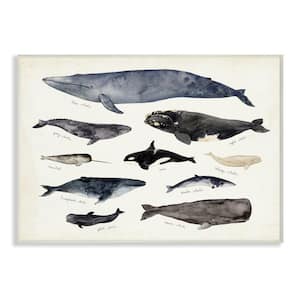The image depicts an educational illustration of various whale species against a white and off-white background, giving it a vintage, postcard-like appearance. There are 10 whales in total, including a large humpback whale at the top, a killer whale in the middle, and a sperm whale at the bottom right. Among these whales are diverse colors, such as gray, black and white, and an all-white beluga whale, which stands out as particularly interesting. The whales are positioned as though they're swimming, without any visible water, enhancing the illustration's focus on their identification rather than their environment. Although the names of the species appear to be written, they are not legible. Overall, it's a detailed and informative depiction designed to help in recognizing different types of whales.